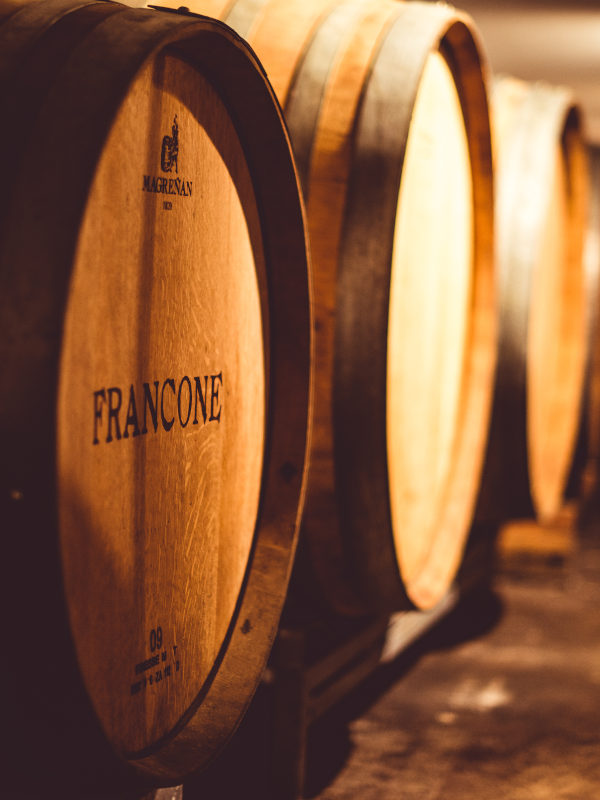The image features three large, weathered wooden barrels, likely used for aging wine or whiskey, arranged in a row against a medium brown wooden wall. The barrels are positioned on an aged wooden floor, adding to the rustic ambiance of the setting. The foremost barrel, crafted from dark brown wood, is clearly marked with "Francone" emblazoned in brown writing, and an emblem at the top that appears to spell "MAGRENAN." Below the brand name, the number "09" is inscribed, though additional details are not fully legible. The barrels in the background are more muted in color, blending shades of brown, beige, and gold, and are less distinguishable. The wooden staves and the metal hoops binding the barrels suggest they have seen extensive use over time.